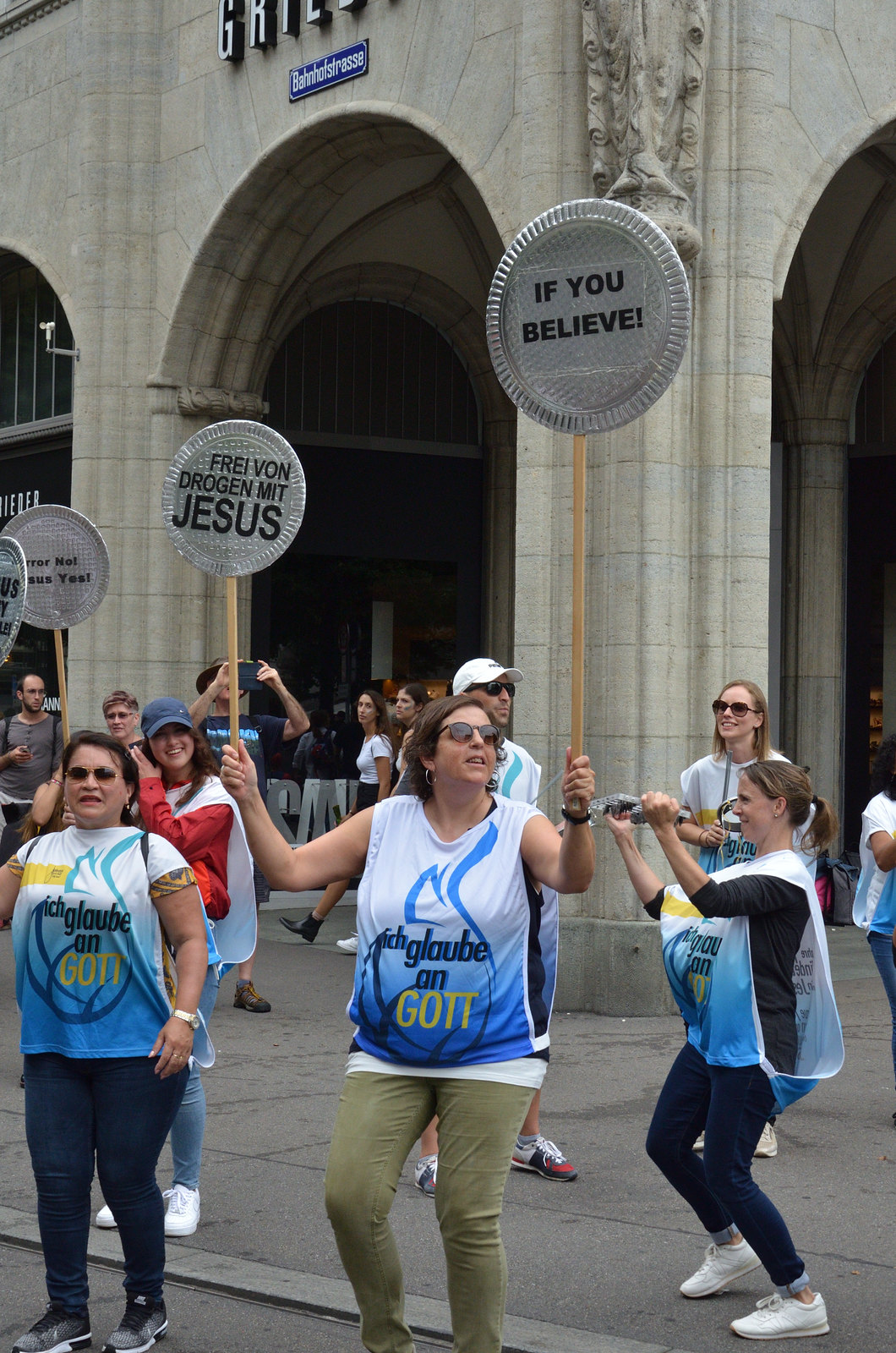The photograph captures a group of individuals standing outside a large stone building with prominent archways. The focal point is a woman in the center, holding two wooden sticks topped with circular pie plates. One plate reads "If you believe!" and the other says "Frau von Drogen mit Jesus." The group members are wearing oversized vests with the words "Ich glaub' an Gott" emblazoned on them. To the left and right of the central figure, other participants also hold similar signs or raise their hands, contributing to a unified display. Spectators in the background can be seen taking pictures with their phones or simply passing by, adding to the lively scene. The atmosphere is slightly overcast, evidenced by the lack of distinct shadows. The entire group seems to be part of a visually engaging public demonstration.